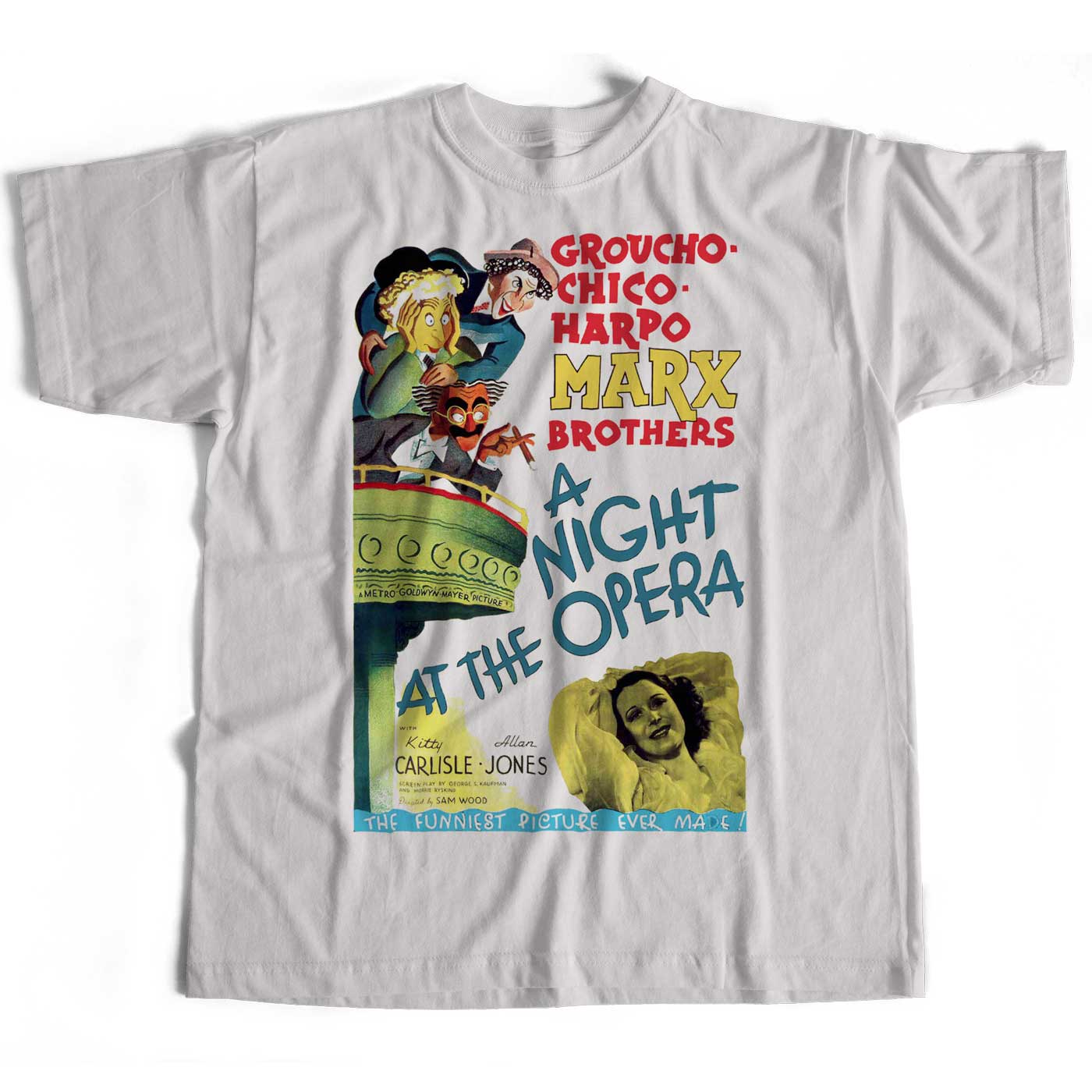The image showcases a white t-shirt displayed flat against a solid white background. The centerpiece is a vibrant and eclectic print featuring both text and images. Prominently displayed in red and yellow text are the names "Groucho, Chico, Harpo, Marx Brothers," and the title "A Night at the Opera." A tagline reads, "The Funniest Picture Ever Made." The names "Kitty Carlisle" and "Alan Jones" are also printed on the t-shirt, with a small note indicating it is "Produced by Sam Wood."

The design integrates both cartoonish illustrations and photographic elements. In the upper left corner, three animated figures – likely the Marx Brothers – peer down from a balcony. One wears a blue jacket and glasses, holding a cigar; another wears a green jacket and a hat, with curly black hair; the third in gray appears to have curly blond hair or another hat. In the lower right corner, a black-and-white photo of a woman with dark curly hair, dressed in flowing clothing and posing with her arms behind her head, gazes back at the viewer – she is identified as Kitty Carlisle.

The overall color scheme of the print includes red, yellow, blue, and black, creating a vivid and nostalgic depiction of the classic film "A Night at the Opera."